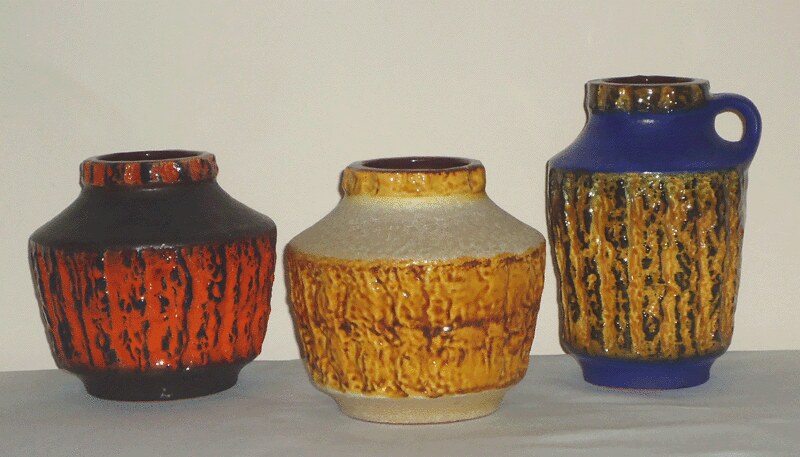This photograph showcases three distinct, hand-thrown pottery pieces arranged in a row on a table against an off-white wall. The pottery, resembling vases, exhibits a harmony in style and texture but varies in shape and color. On the left, a shorter, rounder vase with a crackled surface features a black exterior accented with orange glaze. The central vase, identical in shape to the first, displays a crackled, off-white surface with warm golden brown accents. The vase on the right diverges in shape, standing taller with a jug-like form and a handle. It boasts a golden brown, crackled texture enhanced by blue detailing at the top and bottom. The overall image has a yellow tint, likely caused by the flash during photography.